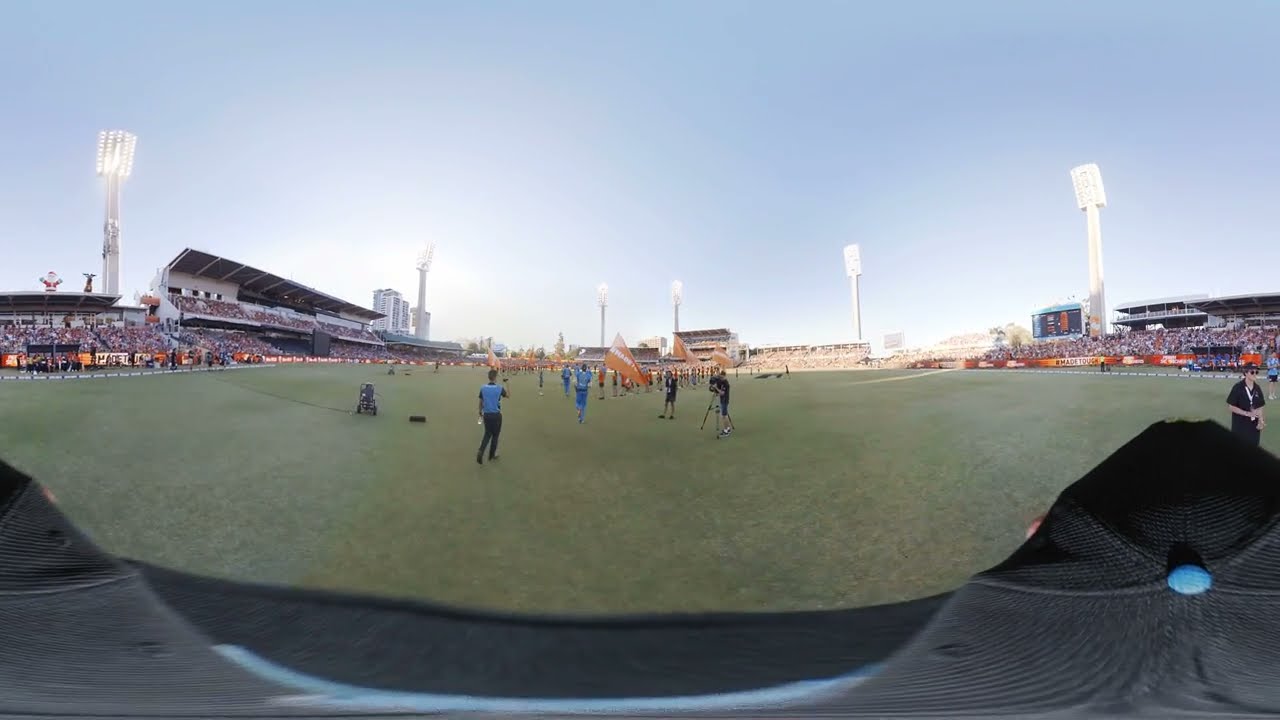This panoramic, fisheye-like distorted image captures the atmosphere of a lively soccer game in a crowded stadium. The foreground prominently features a team of athletes in long-sleeved blue jerseys with black numbers on the back. The jerseys have a red background on which "West" is written in white letters, such as number 28. The players are huddled together on the sidelines, some standing and others sitting on the bench, with a few soccer balls and containers of cold drinks nearby. Coaches or officials, dressed in black, are also visible among them. The expansive green field stretches out to the opposite sidelines, where the opposing team, clad in red or orange uniforms, can be seen. Bright daylight bathes the scene under a clear, sunny sky, emphasizing the excitement building as the game has yet to start.